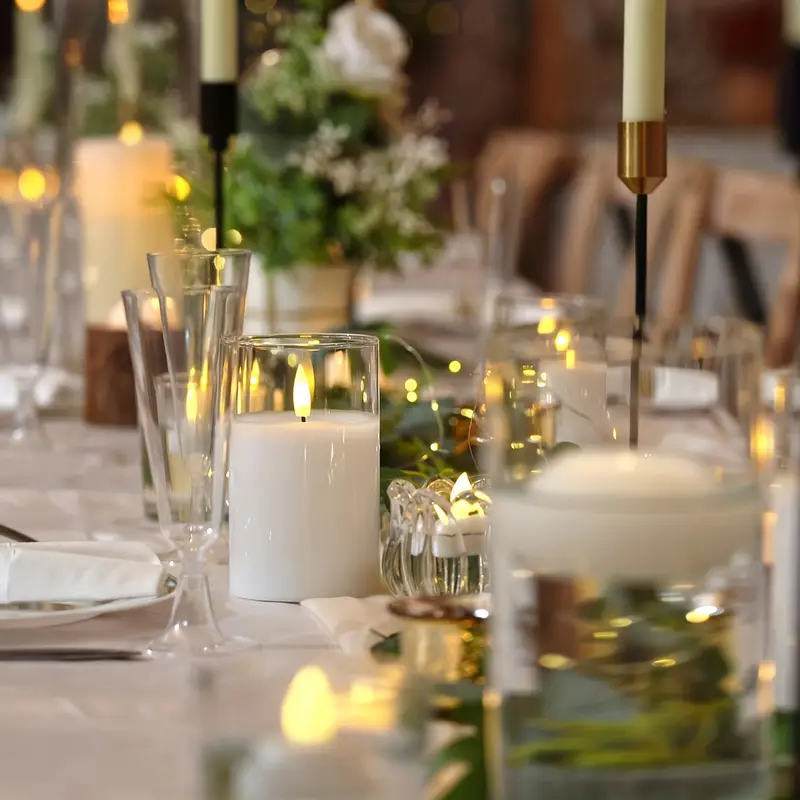This image captures an elegantly set indoor table, likely prepared for a wedding. Centered on the table are green and white flowers arranged in a white vase, amid an array of lit candles. Some are floating in glass jars filled with water while others are housed in brass and black candle holders, one of which is golden and features thin, vertical candles. The table also features wine glasses and white plates, all set against a backdrop of brown walls and wooden chairs. The predominant colors in the photo are white and gold, contributing to the formal and festive atmosphere.